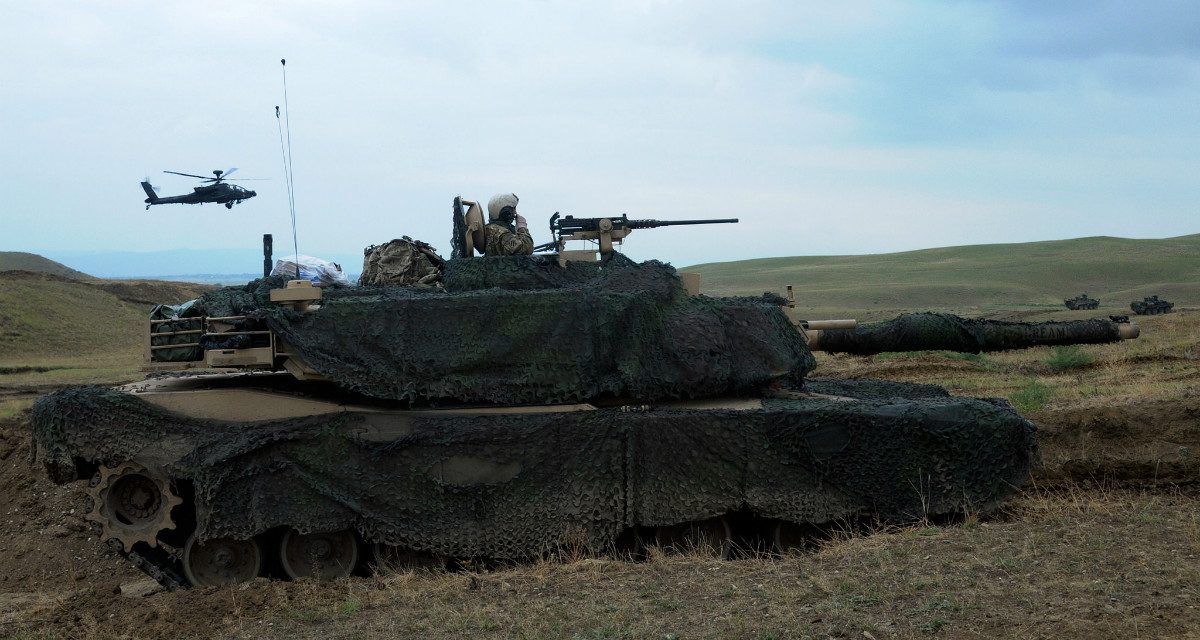This image showcases an M1 Abrams tank positioned in the upper left quadrant of a grassy, hilly battlefield. The tank, facing to the right, is draped in a green, black, and brown camouflage netting. There is a soldier in a camouflaged uniform and a white helmet manning the mounted turret gun. The soldier is holding his hand up to his mouth, appearing to speak into a microphone attached to the helmet. Nearby, an antenna is visible protruding from the tank's gold-colored body. In the background, a helicopter, likely an Apache attack helicopter, is seen flying against a partly cloudy sky comprised of white and blue hues. Two additional armored personnel carriers (APCs) are discernible on the right side of the image, covered in similar black netting. The scene is dominated by a diverse palette of colors including green, blue, white, brown, gray, and black, highlighting the natural elements of the terrain and the sky. The field is characterized by weedy grass and rolling hills, with a log-like shape, identified as part of the tank's camouflage, covering the cannon. Overall, the image conveys a vivid and detailed portrayal of a military scene in action.